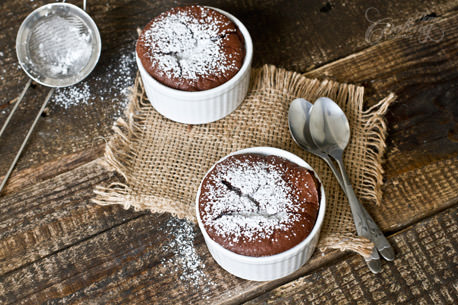This overhead photograph showcases two white ceramic ramekins, each containing a baked item that appears to be a brown cake, possibly a chocolate soufflé, topped with a dusting of powdered sugar. One ramekin is positioned at the top center and the other at the bottom center of the image. The ramekins are set on a rustic brown, knitted cloth which is placed on a dark, textured wooden table, resembling a picnic table with noticeable ridges. To the right of the lower ramekin, there are two silver spoons laying on top of each other in a crossed manner. On the upper left side of the photo, there is a metal sifter, still containing some powdered sugar, indicating that it was used to dust the cakes. A small piece of clove is situated underneath the spoons and the dishes, adding an extra touch of detail to the scene.